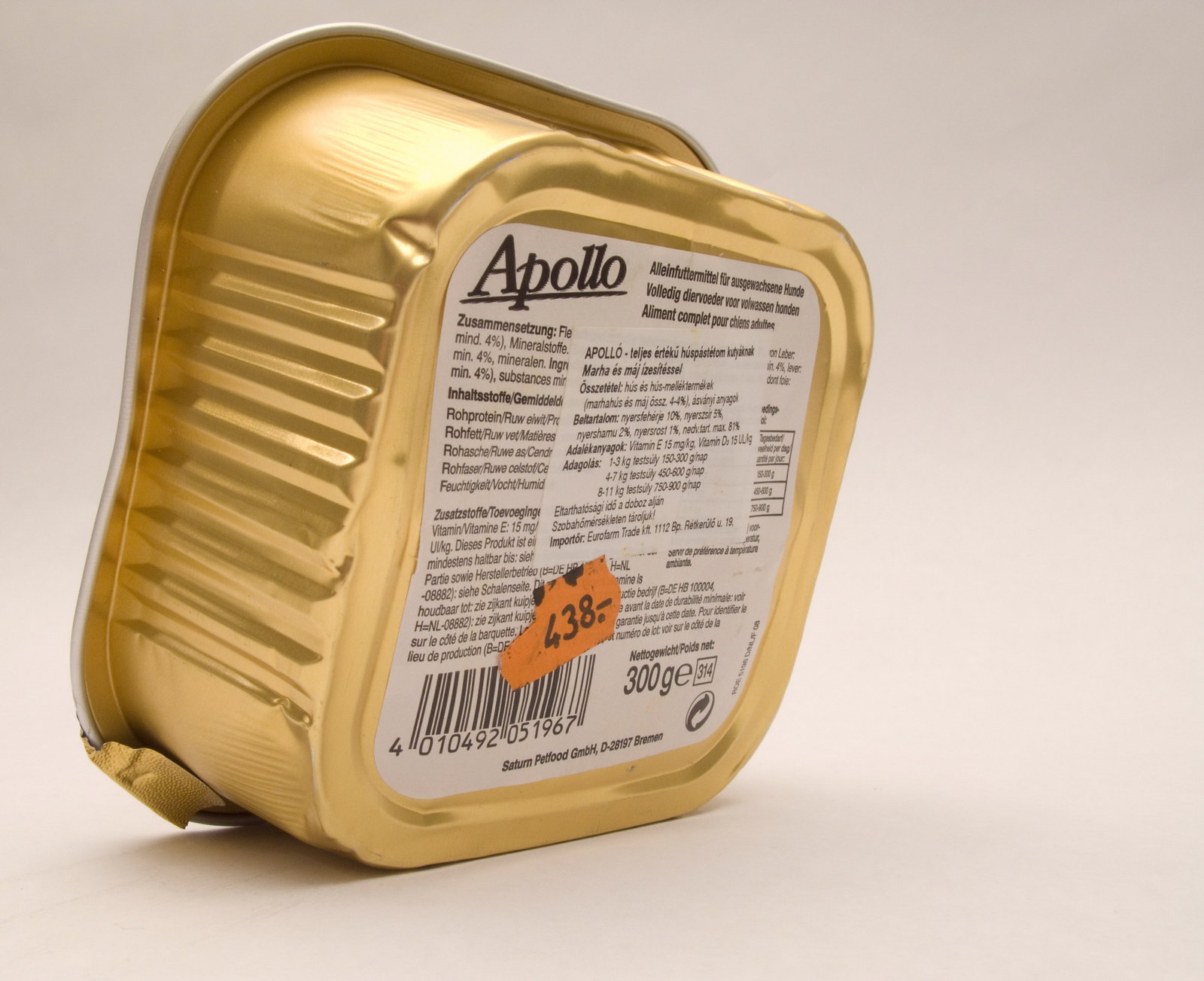The image shows the back of a gold-colored, square metal food container. The container, likely featuring a pull-off foil lid, is possibly for pet food, such as for dogs or cats. Prominently displayed at the top of the back side is a white label with the brand name "Apollo" written in bold black text, underlined. Below this, there is an extensive amount of smaller text believed to be the ingredient list, written in German. Toward the bottom right of the label, the manufacturer information, "Saturn Pet Food GmbH," based in Bremen, is displayed. In the bottom left corner, there is a barcode, and just above it sits an orange price sticker marked with "438" followed by a dash. Additionally, the can is noted to have a net weight of 300 grams.